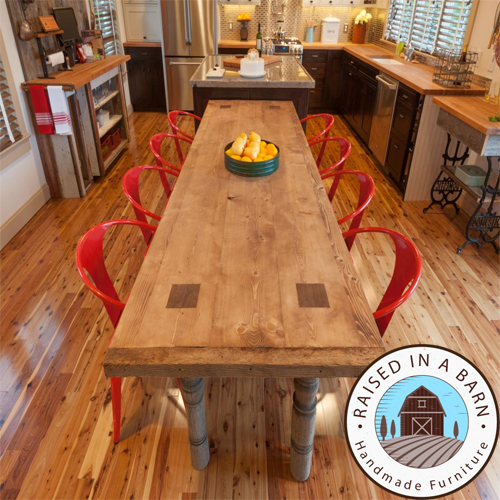This color photograph, presented in a square format, serves as an advertisement for "Raised in a Barn" handmade furniture. Centralized in the image is a long, light brown wooden table with square dark wood insets over the legs at each end, paired with eight modern, low-backed red chairs featuring round chrome arms—four on each side. A round black bowl filled with yellow lemons sits in the center of the table, contrasting starkly with the cream-colored rolls also described.

The backdrop reveals a modern kitchen scene with shiny pine wood laminate flooring. On both sides of the table, countertops and cabinetry share a cohesive wood design, with notable features including a marble island with food items, a cake, a silver refrigerator, a wine cooler, and Venetian-blinded windows. There is a sink and a stove with a brown and white backsplash on the right, flanked by a lamp and kitchen essentials.

In the lower right corner, a logo within a white circle and black border features a barn illustration, framed by trees. The text "Raised in a Barn" arches over the top of the circle, complemented by "handmade furniture" below. This photograph exemplifies the blend of rustic charm and modern design, characterizing the brand's unique handmade furniture offerings.